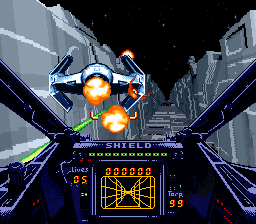This is a high-resolution, square screenshot from a spacecraft shooter video game, captured from the player's cockpit view. Dominating the lower part of the image is the intricate cockpit display. Centrally located on this display, the word "SHIELD" appears prominently in blue, accompanied by several green dots below it, likely indicating shield strength or status. Beneath this, there is a square digital display, surrounded by a series of zeros stretching across the panel with an orange diagram at the far bottom hinting at navigation or targeting information.

In the upper left quadrant of the display, the numbers "0 5" are visible, with contextual blue text above them, possibly indicating ammunition count or another critical statistic. Correspondingly, the bottom right corner features the number "99," similarly accompanied by contextual text above it.

The cockpit's structure also includes small side windows on both the left and right. Through the main windshield at the top, the space outside is visible. Notably, two other spacecraft can be seen outside, one positioned in the far background to the left. This distant spacecraft is under attack, with lasers visibly striking it, and a vivid fireball indicates it's caught on fire.